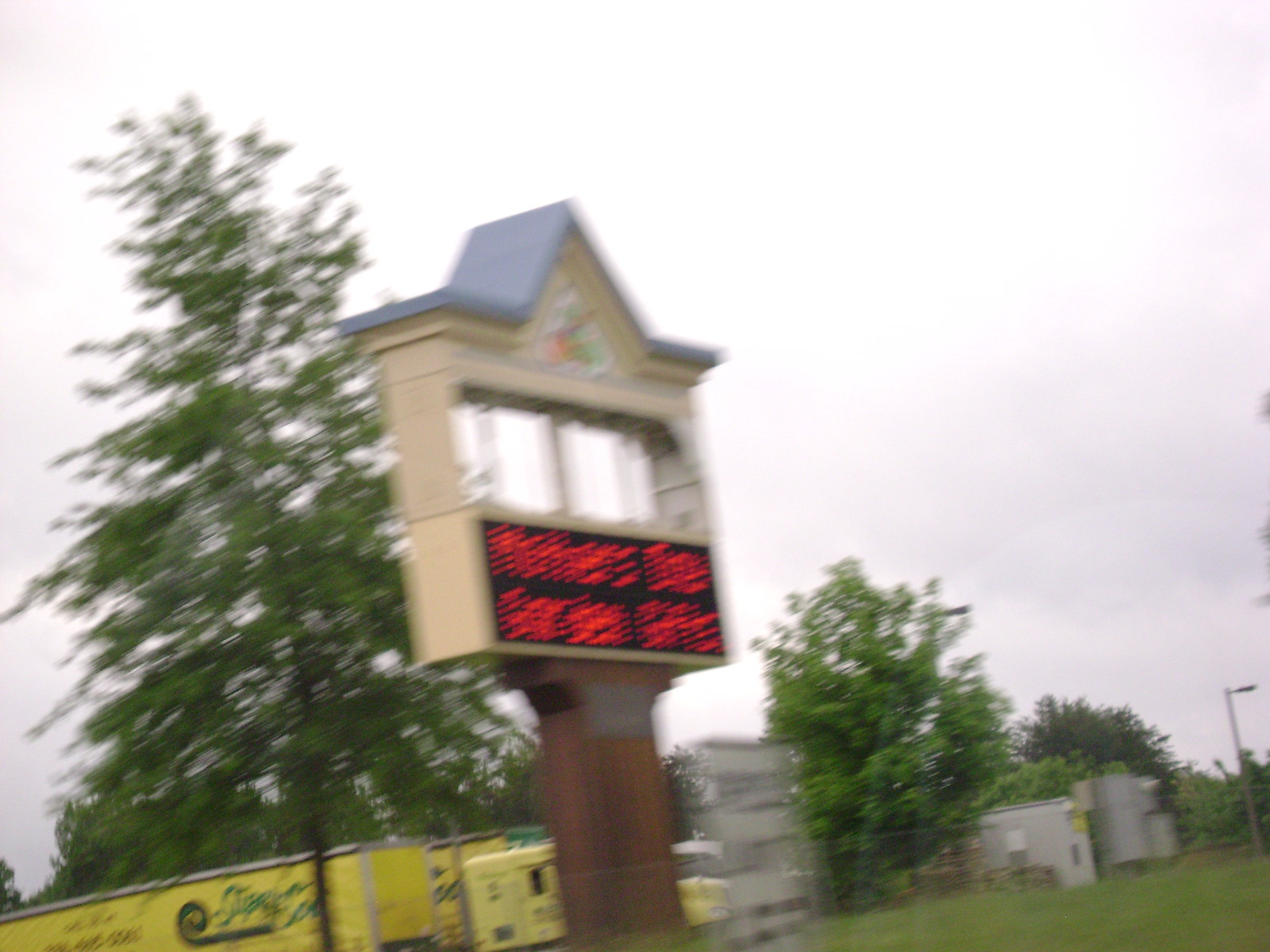The image depicts a slightly blurred photograph of a sign set against a hazy, mostly cloudy sky with some green trees and grass in the background. The sign resembles a small house with a triangular roof and is primarily blue. It features a rectangular, see-through window section that appears partially intact. Below this section, there's a black screen with red text, although the text is too blurry to decipher. The sign is supported by a brown brick or reddish stone pillar. In the background, there's a mix of trees with green leaves, gray buildings, and some vehicles, including yellow trucks with black text. A small portion of a yellow fence is visible in the bottom left corner of the image. The overall setting appears to be near a road with a blend of natural greenery and urban structures.